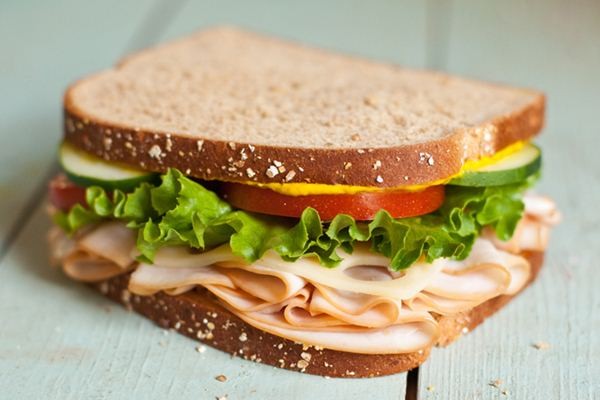This close-up image features a delicious-looking sandwich made with two slices of whole wheat bread, topped with sesame seeds. The sandwich sits on a picnic table made of whitish-gray wood with a slightly blurred background. Inside the sandwich, starting from the bottom, there is a generous amount of thinly sliced deli turkey meat. Above the turkey, there is a slice of Swiss cheese, followed by crisp green romaine lettuce. Sitting atop the lettuce are vibrant red tomato slices and thin slices of cucumber on either side. Finally, the sandwich is finished with a drizzle of bright yellow mustard. The colorful ingredients of the sandwich stand out against the monotone background, capturing a vivid and appetizing scene.